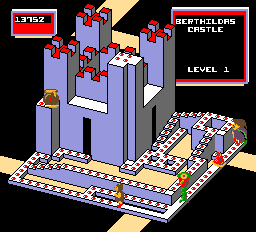In this video game image, the top left corner displays the number "13752." To its right, the text "Birdville's Castle, Level One" is prominently visible next to a black square. The castle depicted is predominantly blue, featuring a black doorway at the bottom and another black doorway on the right. In the top left corner of the screen, there appears to be a brown jar with yellow honey dripping out.

The castle's roof and its towers are adorned with red squares, indicating their flat, cornered tops. At the very bottom of the image, there is a conveyor belt lined with objects that have white tops and red dots. Towards the bottom right of the screenshot, a caterpillar-like creature stands upright next to a red blob. Additionally, a character wearing green attire, including a hood, and displaying red eyes, is also present. The majority of the floor is colored yellow, adding to the vivid and detailed scenery of Birdville's Castle in the game.